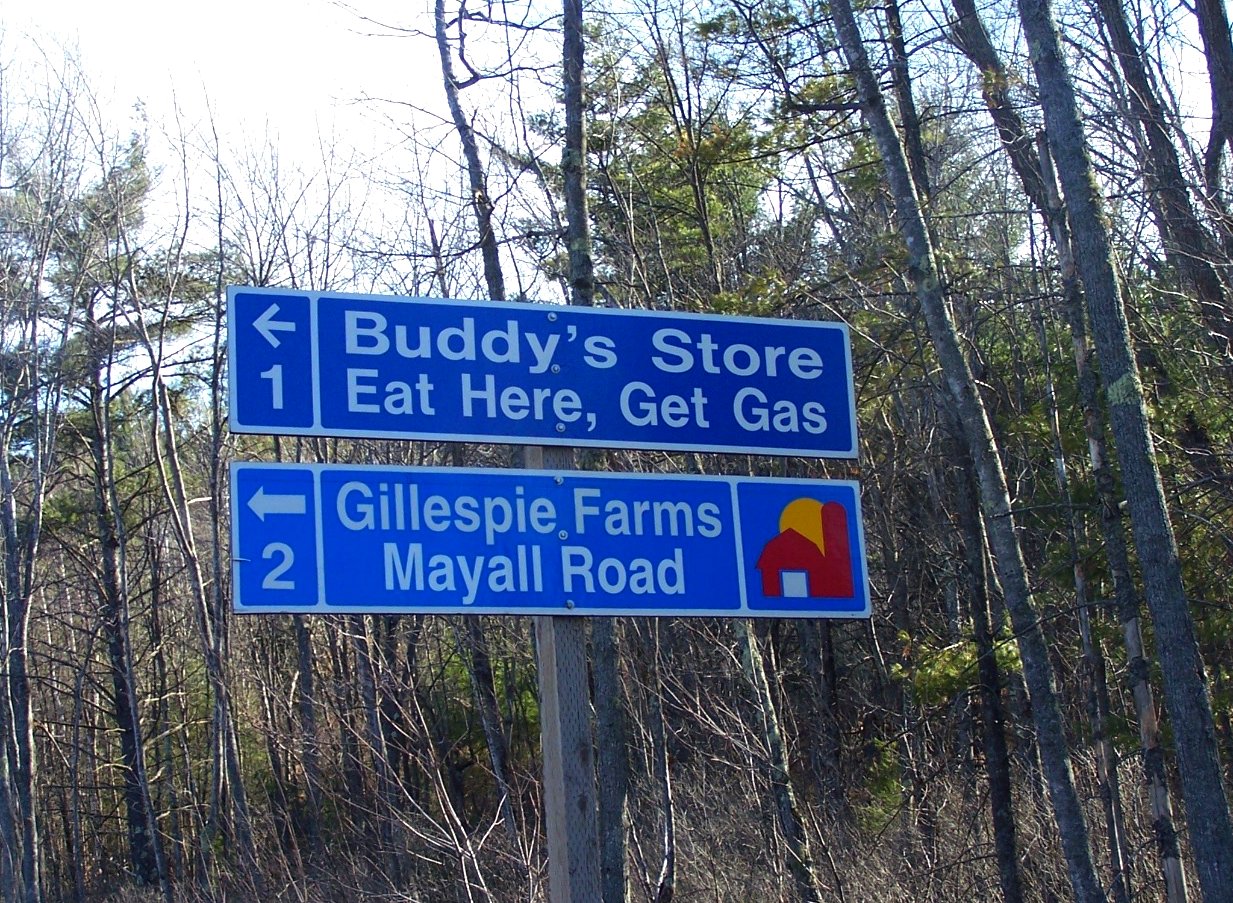In this image, the central focus is on two blue road signs mounted on a silver metal pole. The sky at the top suggests a clear day, and the background reveals a dense forest with mostly bare trees, indicative of winter, interspersed with some fir trees that retain their foliage. The top road sign is a darker blue and features white text that reads "Buddy's Store - Eat Here, Get Gas" with the number "1" and an arrow pointing right. The bottom sign is a lighter blue, also with white text, stating "Gillespie Farms - Mayall Road," next to the number "2" and another right-pointing arrow. This sign includes a small icon of a red barn set against a backdrop of a yellow sun. The forested background with its mix of brown tree trunks and green fir trees suggests a rural mountainous area.